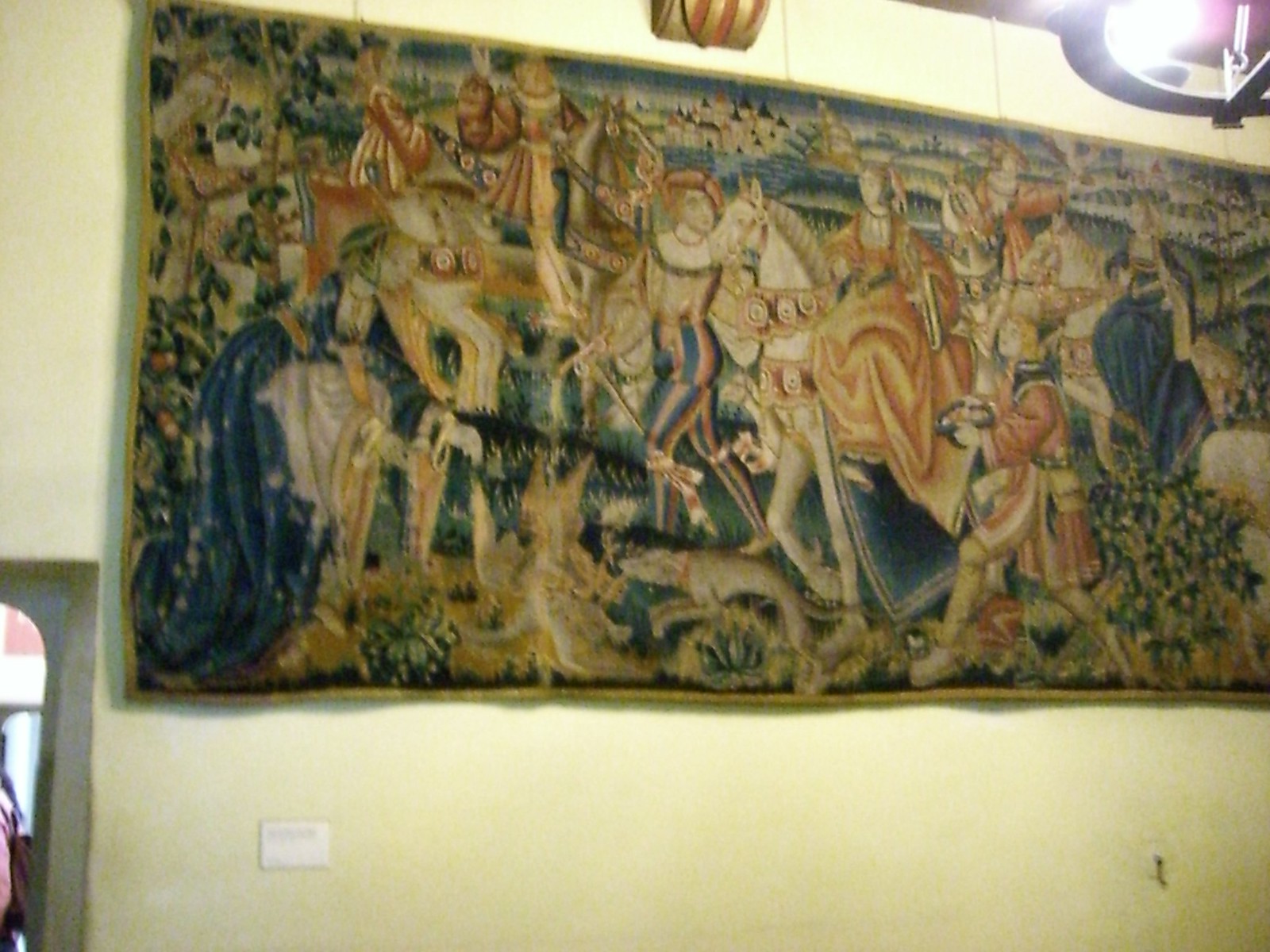This color photograph, taken indoors, centers on a very large tapestry hanging on a cream-beige wall, occupying the majority of the space. In the top right corner, a bright light fixture illuminates the tapestry, suggesting it could be displayed in a museum setting. The tapestry depicts a detailed medieval scene, characterized by a sense of royal presence and historical significance. At the heart of the scene, a regal figure presumed to be a princess, dons a large dress while seated on a magnificently adorned white horse. Surrounding her, various men appear in period-specific garments, including bloomers and ruffled shirts, hinting at their noble status. A king is depicted kneeling before the princess, engaged with objects on the grass, adding to the sense of a royal narrative. The scene includes ample greenery and a distant view of a castle, enhancing the medieval ambiance. The tapestry's faded yet rich palette integrates basic colors like blues, greens, reds, white, and yellow, all contributing to its visually arresting portrayal of historical grandeur.